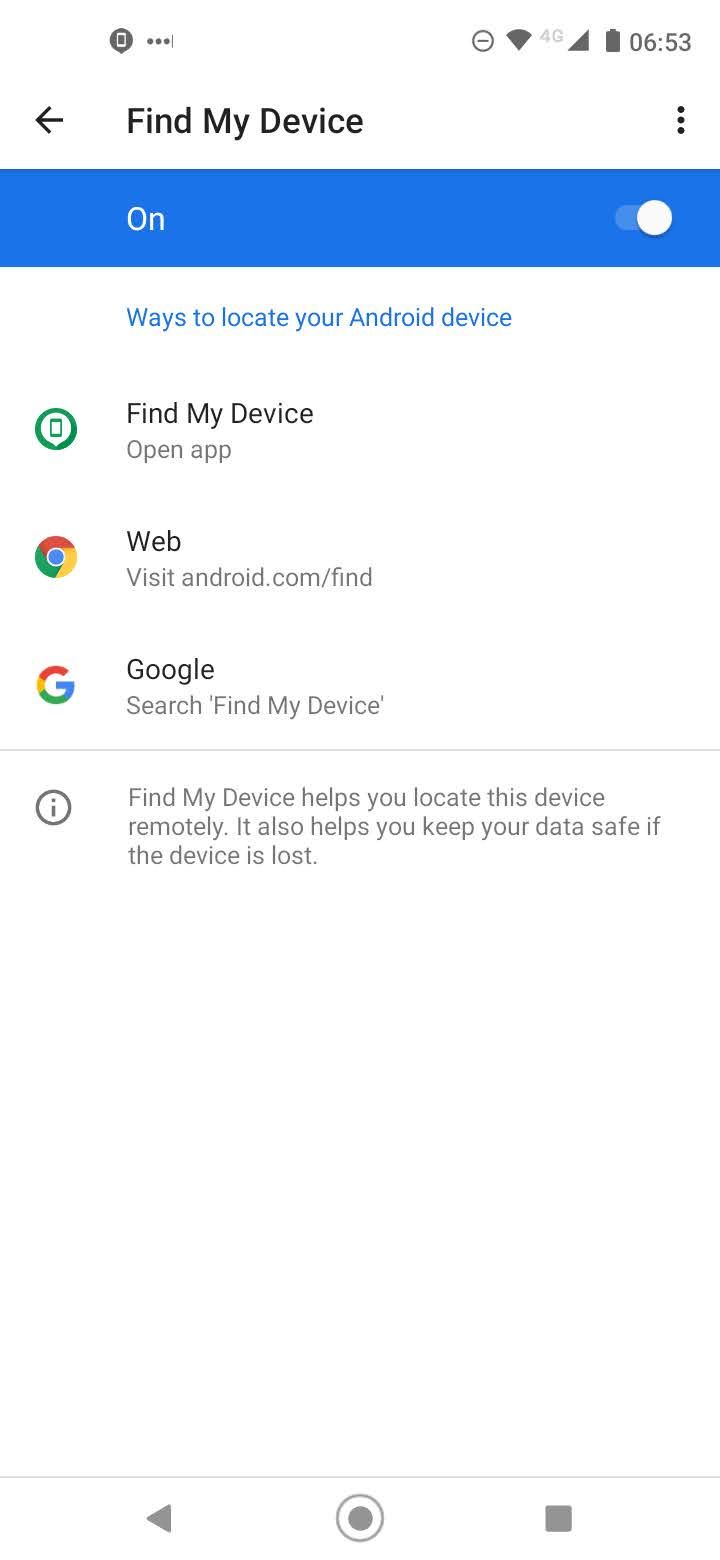The image depicts a smartphone screen displaying the 'Find My Device' feature. At the very top, the status bar is visible, showing the time as 06:53 in military format, alongside battery life, Wi-Fi, and 4G indicators.

Below the status bar, a prominent header reads 'Find My Device.' An arrow points to the left of this header. Directly under the header, there is a blue bar with the word 'ON' in white text, accompanied by a slider button currently positioned to the right, indicating that the feature is activated.

Further down, the text 'Ways to locate your device' is shown in blue, followed by several options for finding the device. The first option reads 'Android Device' in blue text with a 'Find My Device' label beneath it. To the left of this label is a green circle icon featuring a green device symbol in the center.

The second option instructs users to visit 'android.com/find' and is paired with a Google Chrome icon to the left. The text 'Web' accompanies this option.

The third option invites users to search 'Find My Device' on Google, with a multicolored 'G' logo to the left. Below this, there's a brief description: 'Find My Device helps you locate this device remotely. It also helps you keep your data safe if the device is lost,' accompanied by an information icon to the left.

At the very bottom of the screen are three navigation icons: a back button, a solid circle with another circle around it, and a square. The overall background of the screen is white.